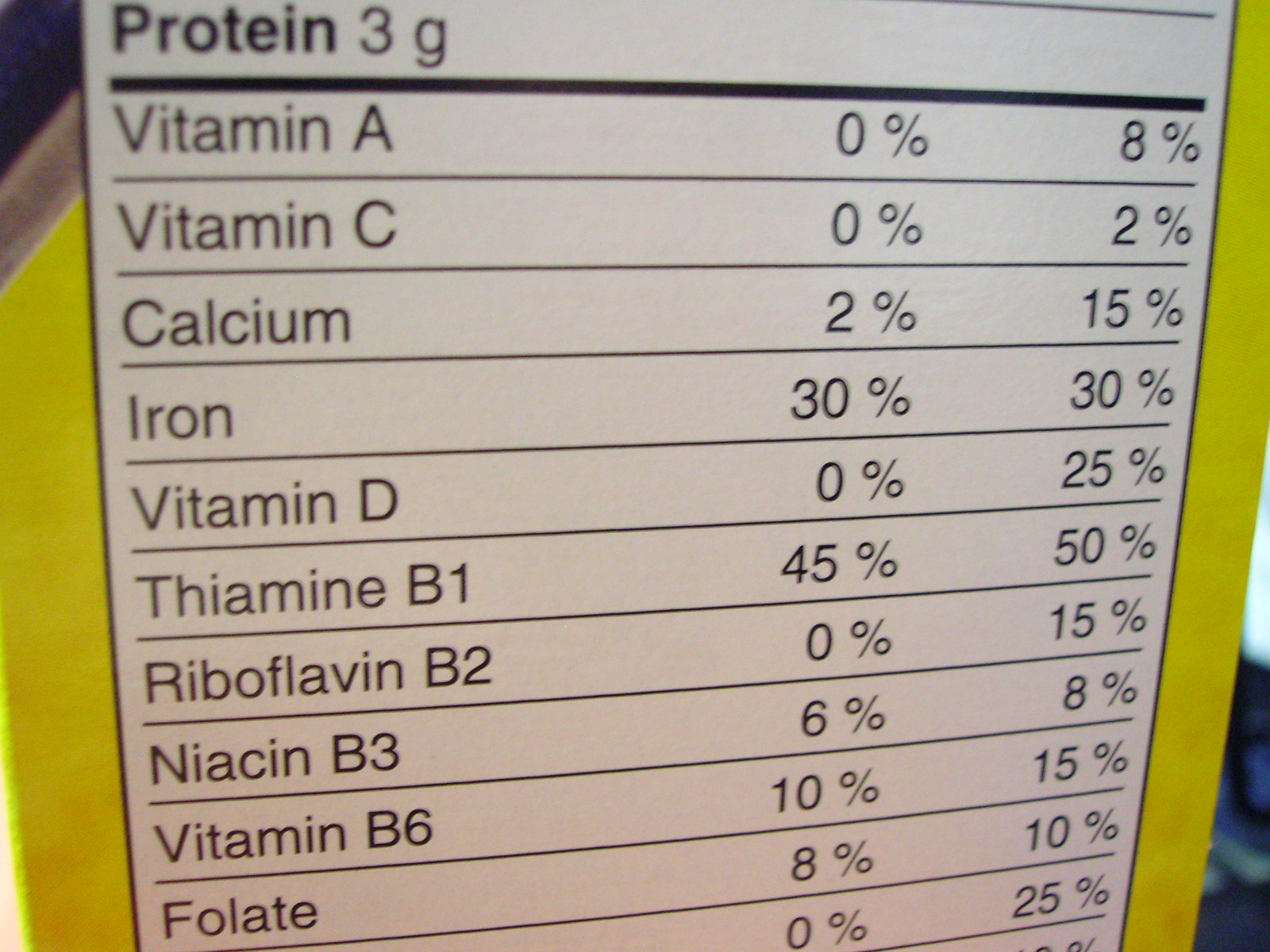The image features a detailed nutrition label bordered in yellow, with a black section in the top left corner. The label indicates the following nutritional content:

- **Protein:** 3 grams
- **Vitamin A:** 0% of the Daily Value (DV)
- **Vitamin C:** 0% DV and 2% DV
- **Calcium:** 0% DV and 50% DV
- **Iron:** 30% DV and another listing of 30% DV
- **Vitamin D:** 0% DV and another listing of 12% DV
- **Vitamin B1 (Thiamin):** 0.5% DV and 3% DV
- **Vitamin B2 (Riboflavin):** 0% DV and 50% DV
- **Niacin (Vitamin B3):** 6% DV and 8% DV
- **Vitamin B6:** 10% DV and 50% DV
- **Folate:** 8% DV, 10% DV, and a third listing of 0%

The label meticulously breaks down the percentages of daily vitamins and minerals, with some entries showing multiple values, demonstrating the varying levels of these nutrients in different servings or different components of the item.